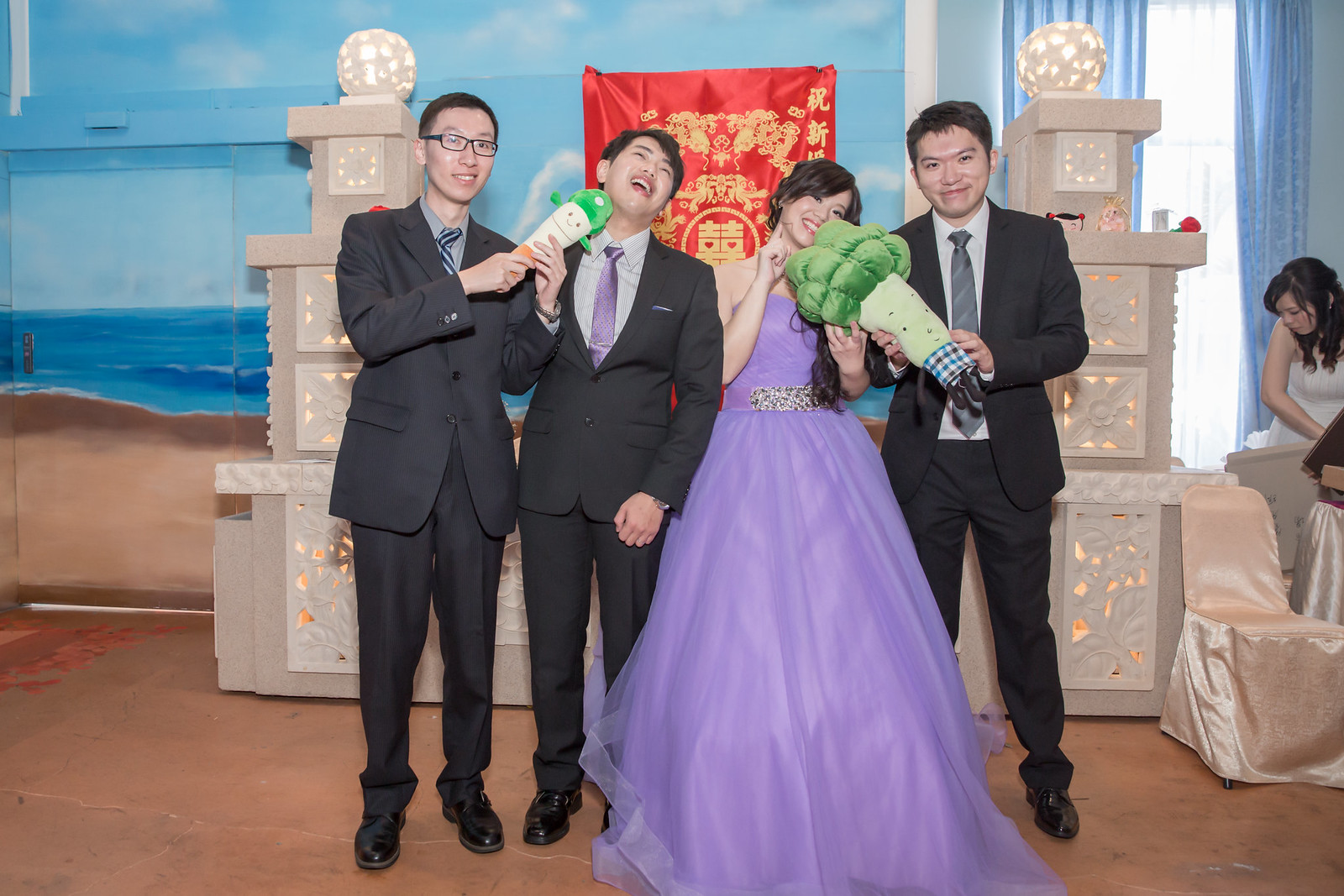This photograph appears to capture a special event, possibly a wedding or ceremony, featuring four Asian individuals on a stage with decorative props. Three men and one woman stand together, all dressed in formal attire. The three men are in black suits with distinctive ties: the man on the left wears a blue-striped tie and glasses, the man on the right in an unbuttoned jacket sports a black tie, while the man second from the left dons a purple tie that matches the woman's long lavender dress. The woman, who is holding a stuffed broccoli, stands next to the man with the purple tie, who is laughing with his head thrown back, and beside him is another man holding a toy cloth microphone with green hair up to his mouth. The backdrop features a painted beach scene with sand, water, waves, and cloudy blue skies, along with a prominent red satin or silk cloth, possibly with Chinese writing. There are white pedestals with glowing white balls, silk-covered chairs, and additional people in formal attire in the background. The floor appears to be made of orange-colored stone.